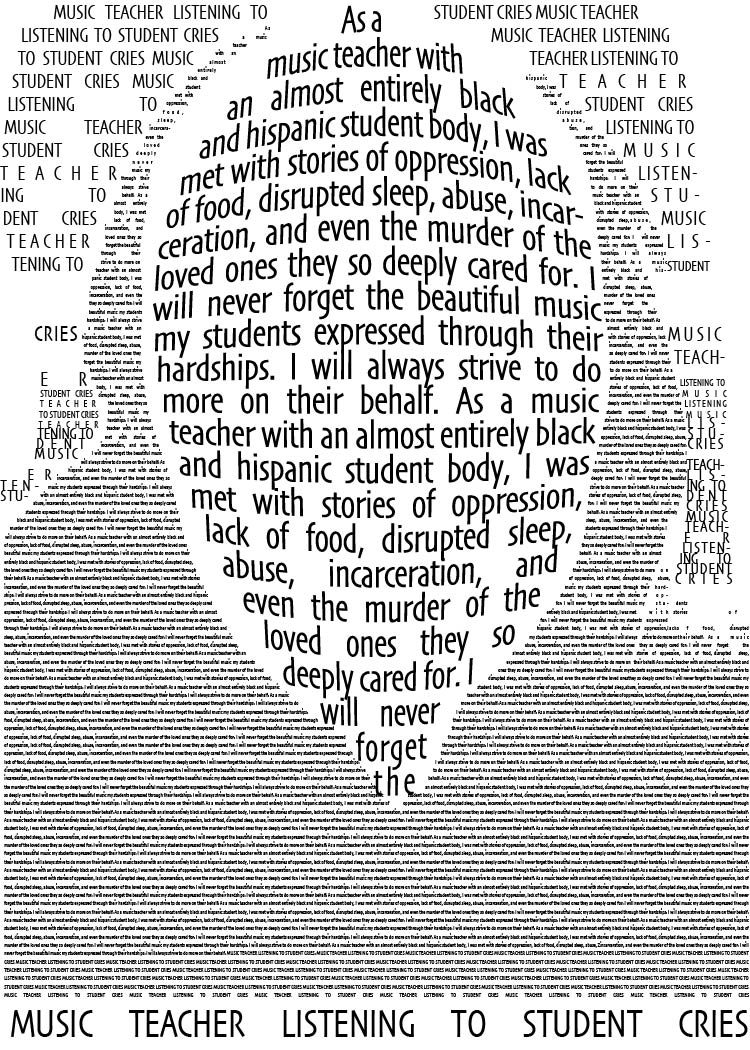The image is a black-and-white piece of text-based artwork centered around the experiences of a music teacher. The text, which fills the entire image, is meticulously arranged, with some parts written so small they blend into the background to create a grayish tone. In contrast, large, bold black letters in the center form the shape of a teardrop or balloon. These prominent words read, "As a music teacher with an almost entirely black and Hispanic student body, I was met with stories of oppression, lack of food, disrupted sleep, abuse, incarceration, and even the murder of loved ones they so deeply cared for. I will never forget the beautiful music my students expressed through their hardships. I will always strive to do more on their behalf." Beneath this poignant declaration, the smaller text at the bottom completes the narrative: "music teacher listening to student cries." The overall design resembles a face, with the expressive and detailed text combining to create a powerful visual and emotional impact.